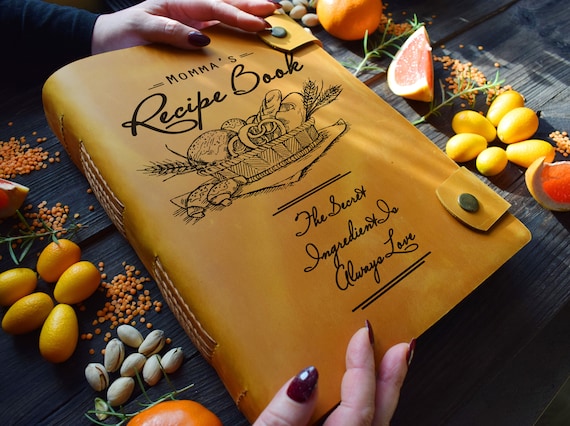A detailed photograph captures a beautifully crafted leather-bound cookbook titled "Mama's Recipe Book." The book, made of yellow or light brown leather, features a sophisticated cover design with etched illustrations, including a detailed bread basket with croissants and wheat stalks. The title "Mama's" appears in small print, while "Recipe Book" is elegantly scripted. Below the illustration, a heartfelt phrase reads, "The secret ingredient is always love," also in cursive script.

The cookbook is carefully held by a pair of hands with crimson red, acrylic-pointed nails, giving the impression of a woman's hands. These hands, positioned at the book's edges, suggest a tender and cherished grasp. The leather cover is secured with two buttoned latches on the sides, emphasizing its premium craftsmanship.

The book rests on a dark brown, rough-hewn wooden table, partially concealed by an assortment of culinary ingredients. Surrounding the cookbook are sections of orange, pistachios, rosemary, small golden plum-style tomatoes, and seeds, hinting at the diverse flavors contained within its pages. The overall composition exudes a sense of warmth, tradition, and culinary love.